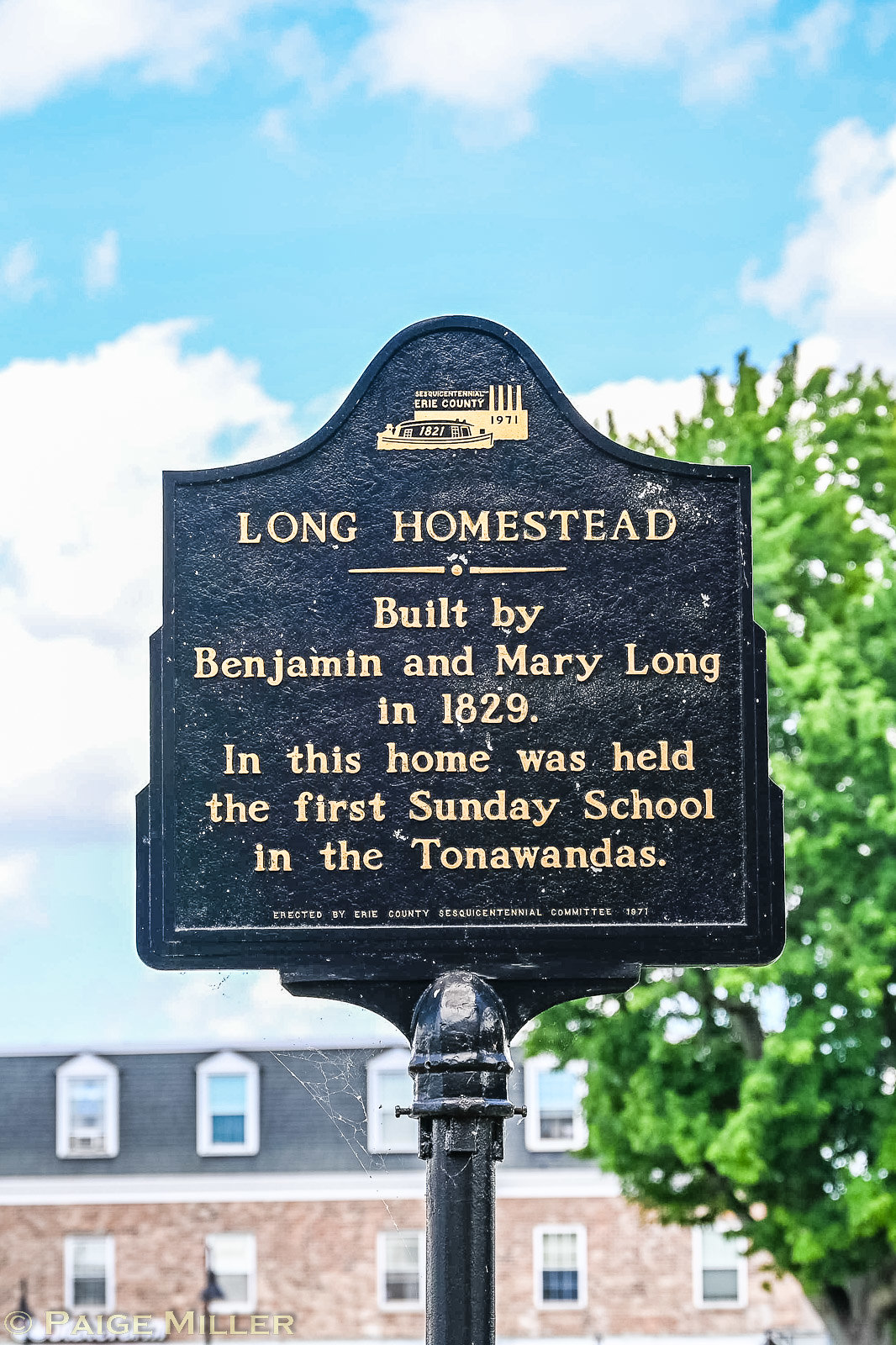This photograph features a black metal sign with prominent yellow text at the top. The sign displays a logo that appears to say "Erie County 1971," accompanied by images of a large ship and a smaller tugboat marked "1828." Below this logo, in yellow letters, it reads "Long Homestead, built by Benjamin and Mary Long in 1829." The text continues to state that this home hosted the first Sunday school in the Tonawandas. In small white letters, it mentions "erected by Erie County committee in 1871," although some of these details are difficult to decipher. 

The sign is mounted in front of a green tree and a wide brick building with a black roof and approximately 10 white windows. Additionally, there's a spiderweb visible on the left side of the post supporting the sign. The tree is positioned to the right of the sign in the photograph.